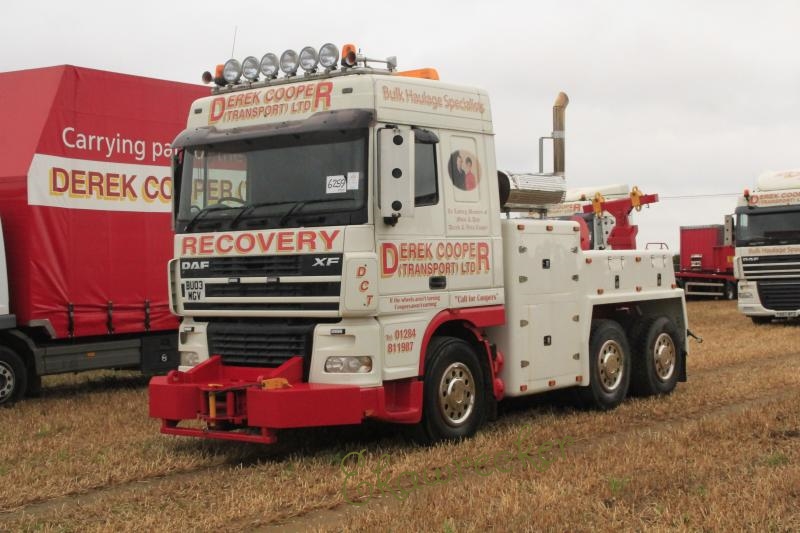The image depicts a white recovery truck, likely a tow truck specialized for pulling other vehicles, such as trucks or semis, out of ditches and breakdown situations. The truck features prominent red lettering. Just below the windshield, it reads "Recovery," indicating its purpose. On the side, the branding "Derrick Cooper Transport LTD" is boldly displayed, accompanied by the phrase "Bulk Haulage Specialists" at the top. The cab door showcases a circular image of two individuals, presumably Mr. Derrick Cooper and a companion. The truck has a distinctive red front bumper, designed for towing. It is parked on a grassy dirt road, with another similar vehicle visible behind it, and additional trucks with red covers marked with the same company name in the background, suggesting a fleet used by Derrick Cooper Transport LTD for recovery and haulage operations. The truck's rear equipment, though not entirely clear, seems to involve locking mechanisms for securing loads or tow lines.